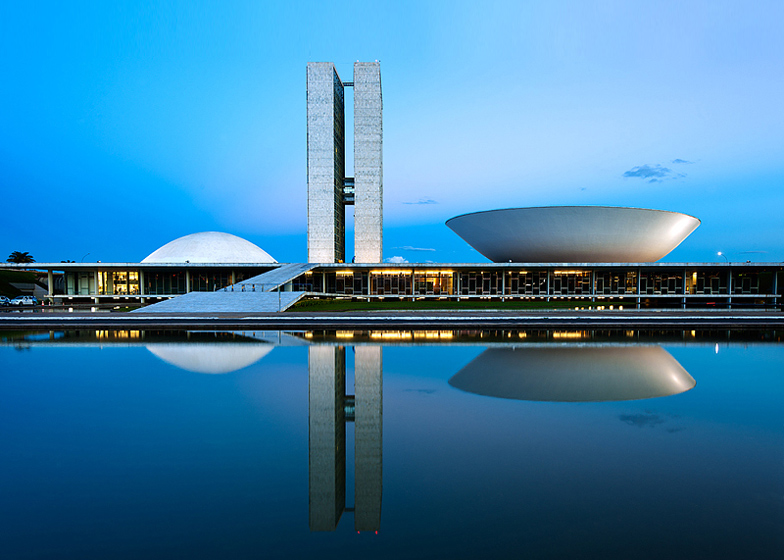The image depicts a modern, architecturally unique building complex situated beside a reflective body of water, possibly a pond or reservoir. The main structure is a long, possibly one or two-story building, reminiscent of a warehouse or concourse you might find at an airport, characterized by its linear design and illuminated interior lights. Sitting atop this structure is an enormous, metallic bowl-shaped installation, which could easily be mistaken for a piece of contemporary art. Adjacent to this, on the left side, is a large inverted dome or a bowl turned face down, contributing to the distinctive skyline. Dominating the central portion of the scene are two high-rise, rectangular towers, seemingly connected by several skybridges, which rise dramatically and resemble twin pillars. These towers lack visible windows on the side facing the viewer, further adding to the mystery of their function. The entire scene is captured under a clear blue sky with scattered clouds, and the complex is framed by a few trees in the distance. Importantly, this entire composition is reflected perfectly in the tranquil water at the foreground, creating a mirrored double of the striking architectural forms. The serene and surreal quality of the image raises questions about whether it is a photograph of a real place or a digitally created scene.